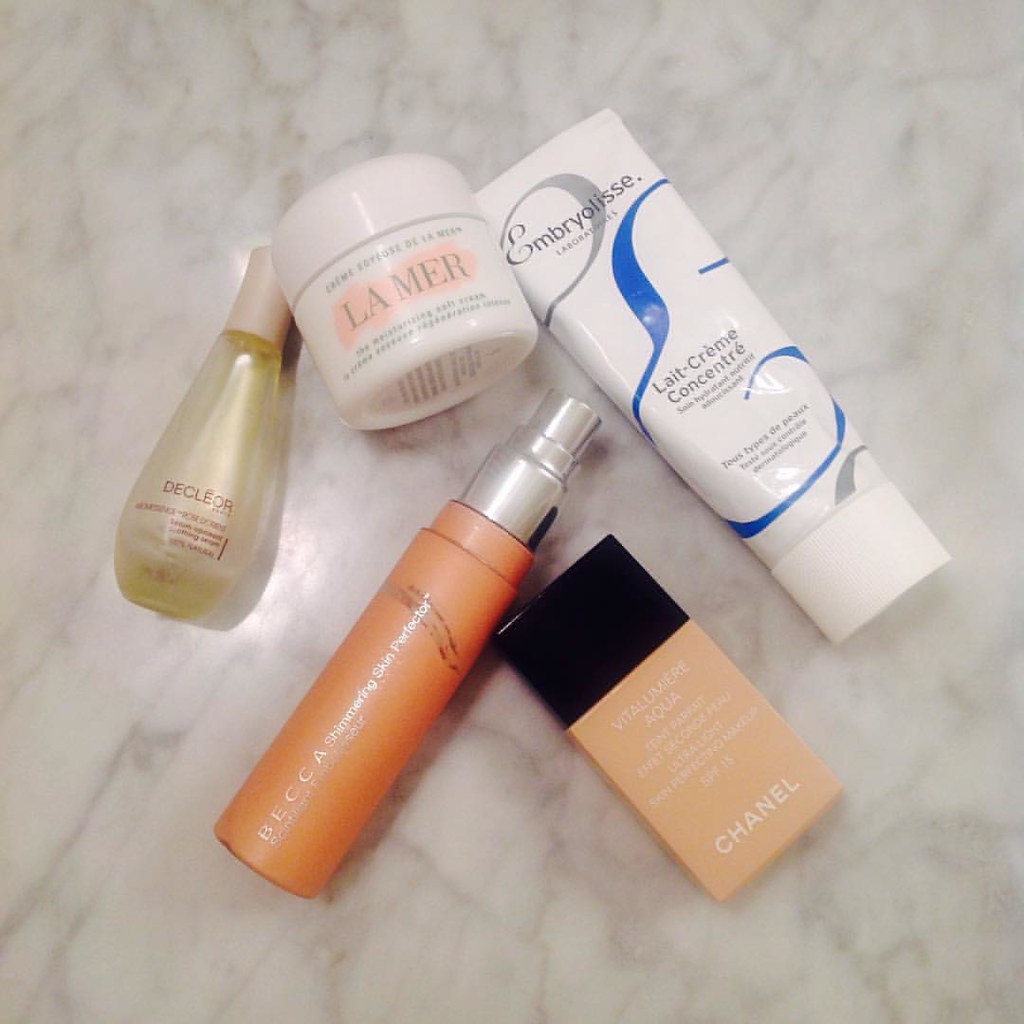**Caption:** 

A meticulously arranged selection of luxurious beauty products is displayed on a pristine white marble surface, illuminated by soft indoor lighting that casts a gentle reflection in the center-left of the image. The collection includes five distinct items:

1. A slender, pear-shaped bottle with a beige cap, containing a yellow liquid labeled "Decléor".
2. A short, cylindrical skin cream jar with a rounded white cap, adorned with the "La Mer" logo set against a subtle pink background.
3. A long tube featuring a white cylindrical cap at the bottom, decorated with blue and gray curls, branded with "Embryolisse Lait-Crème Concentré".
4. An orange spray bottle resembling the color of a carrot, topped with a silver push-down cap, marked "Becca".
5. A flat, rectangular prism-shaped container, with a bottom portion in a delicate pink hue and a large, flat black square cap, labeled "Chanel".

The carefully curated assortment of products exudes sophistication and elegance, perfect for a high-end beauty regimen.